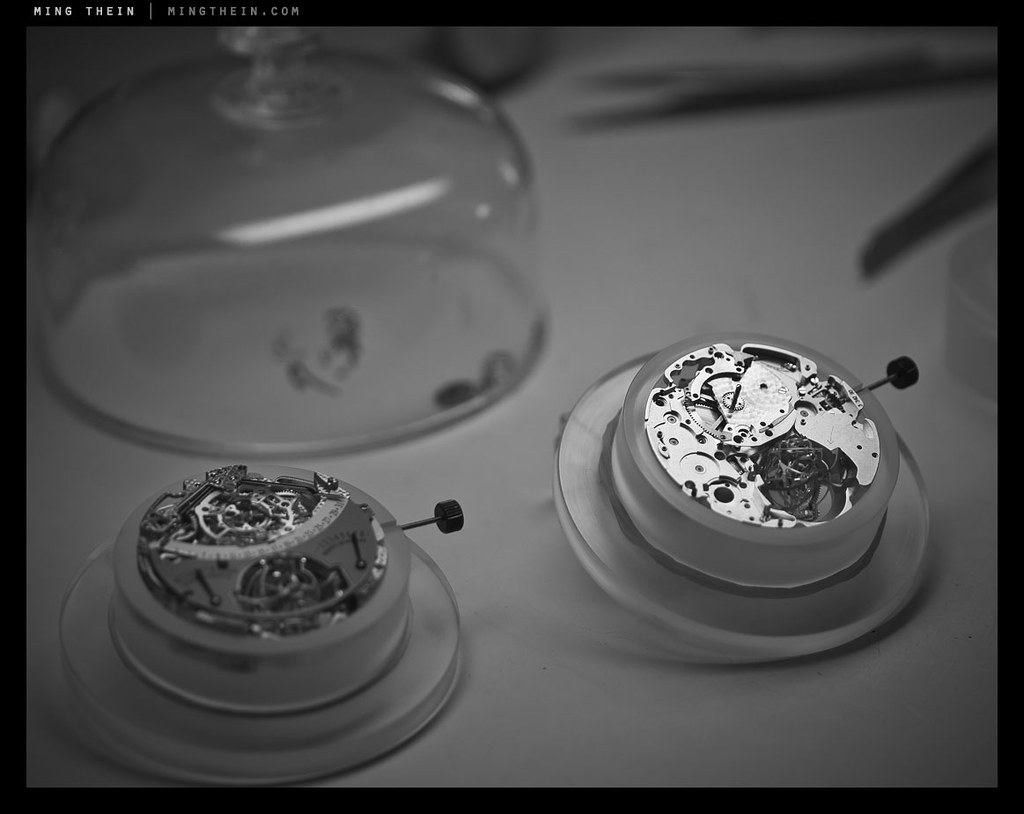The black and white image captures two vintage, circular mechanical devices partially disassembled to reveal their intricate inner workings. These devices, possibly clock mechanisms, expose gears, wheels, screws, and winding keys on their right side, inviting interaction through twisting to set them in motion. They are carefully placed on what appears to be a white table cover, suggesting a repair or examination scene. A partially visible tool in the upper corner hints at ongoing work. Above these devices, a round glass jar with a knob sits, adding to the vintage aesthetic and indoor setting. The photograph, slightly blurred in some areas but sharply focused on the primary subjects, presents a meticulous study of the delicate craftsmanship of bygone technologies.